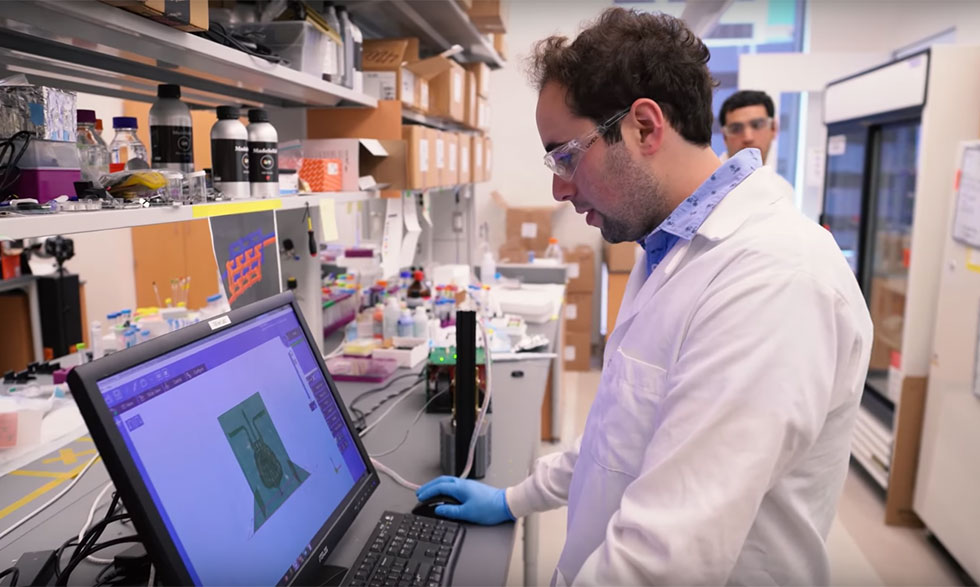The photograph shows the interior of a cluttered laboratory or clean room. In the foreground, a scientist in a white lab coat and blue polka-dotted shirt is operating a computer with his right hand on a mouse. This scientist is wearing blue latex gloves, safety goggles, and has short, slightly disheveled dark hair with a receding hairline, and stubble. He is focused on the computer screen, which displays a central greenish pattern. Behind him, another scientist is partially visible, peering over from the background. This second scientist, also with dark hair and wearing safety goggles, stands near a large window or display case. The workspace is narrow and packed with various scientific supplies—white shelves laden with bottles, vials, test tubes, sampling pipettes, and cardboard boxes with unlabeled contents. Despite the detailed view of the environment, nothing specific identifies the exact type of research or technology they are engaged in.